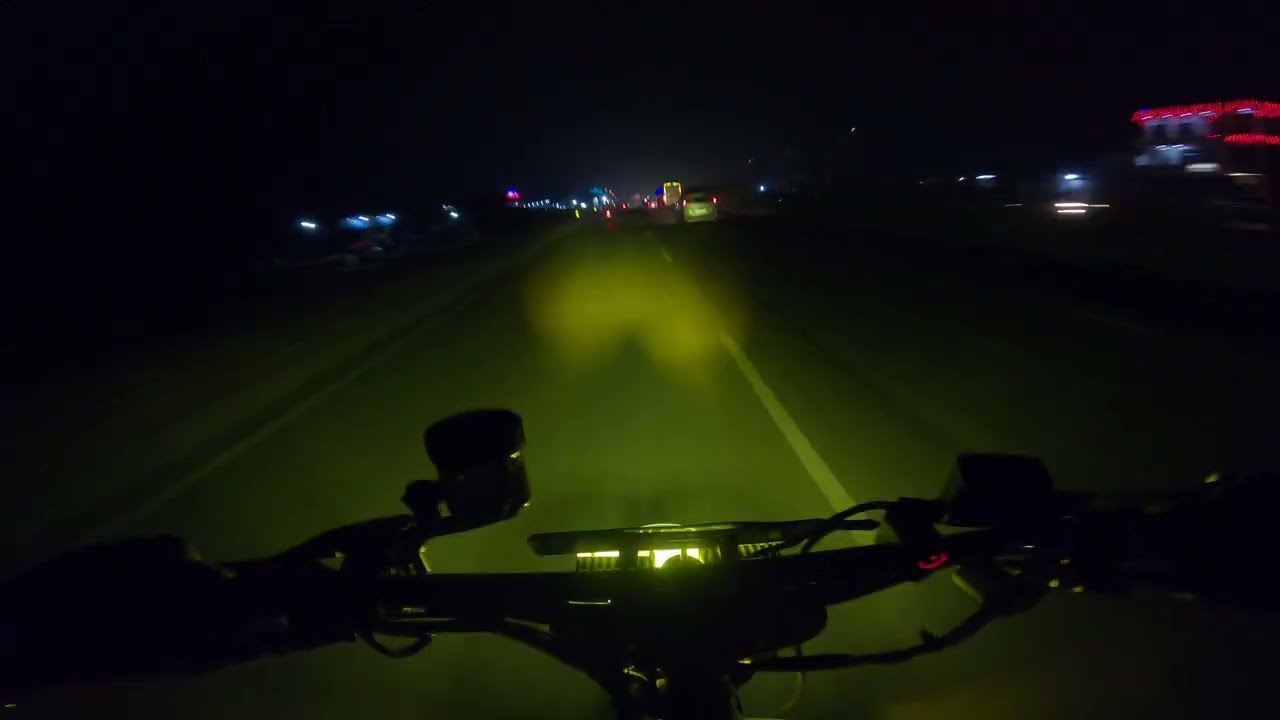In this nighttime scene, the blurry photo captures the perspective of someone traveling down a road, likely on a bicycle or motorcycle. The foreground is illuminated by the yellow headlight, casting a glow onto the road ahead. The road is marked with white lane stripes extending into the distance. Traffic flows above on an overpass, indicated by faint brake lights and various colored lights above and ahead. The blurred surroundings suggest an urban or industrial area, highlighted by illuminated buildings, including one with distinct red lights on the right. A few stars are faintly visible in the night sky, and scattered street and traffic lights contribute to the ambient glow of this bustling, nocturnal setting.